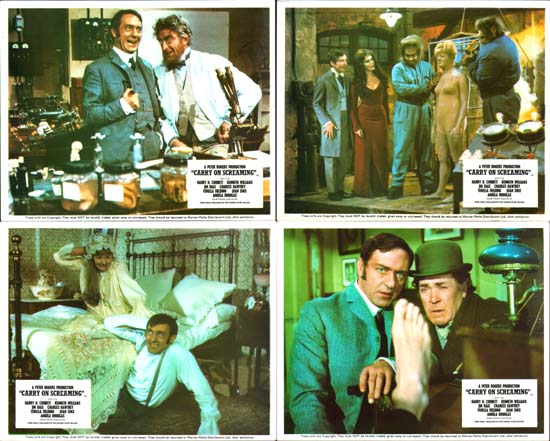The image displays four stills from what appears to be a humorous or dark comedy titled "Carry On Screaming." The top left photograph shows two men dressed in suits conversing in a kitchen, with three jars of food and two forks on the countertop between them. The top right image depicts five individuals performing on a stage, seemingly part of the same production. In the bottom left, a woman in a nightgown sits on a bed and appears to be beating a man emerging from underneath it. The bottom right picture features two men, one in a gray suit and the other in a brown coat and top hat, intently looking at a bare right foot extended towards them. Each image contains text boxes in the corners, reinforcing the "Carry On Screaming" theme.